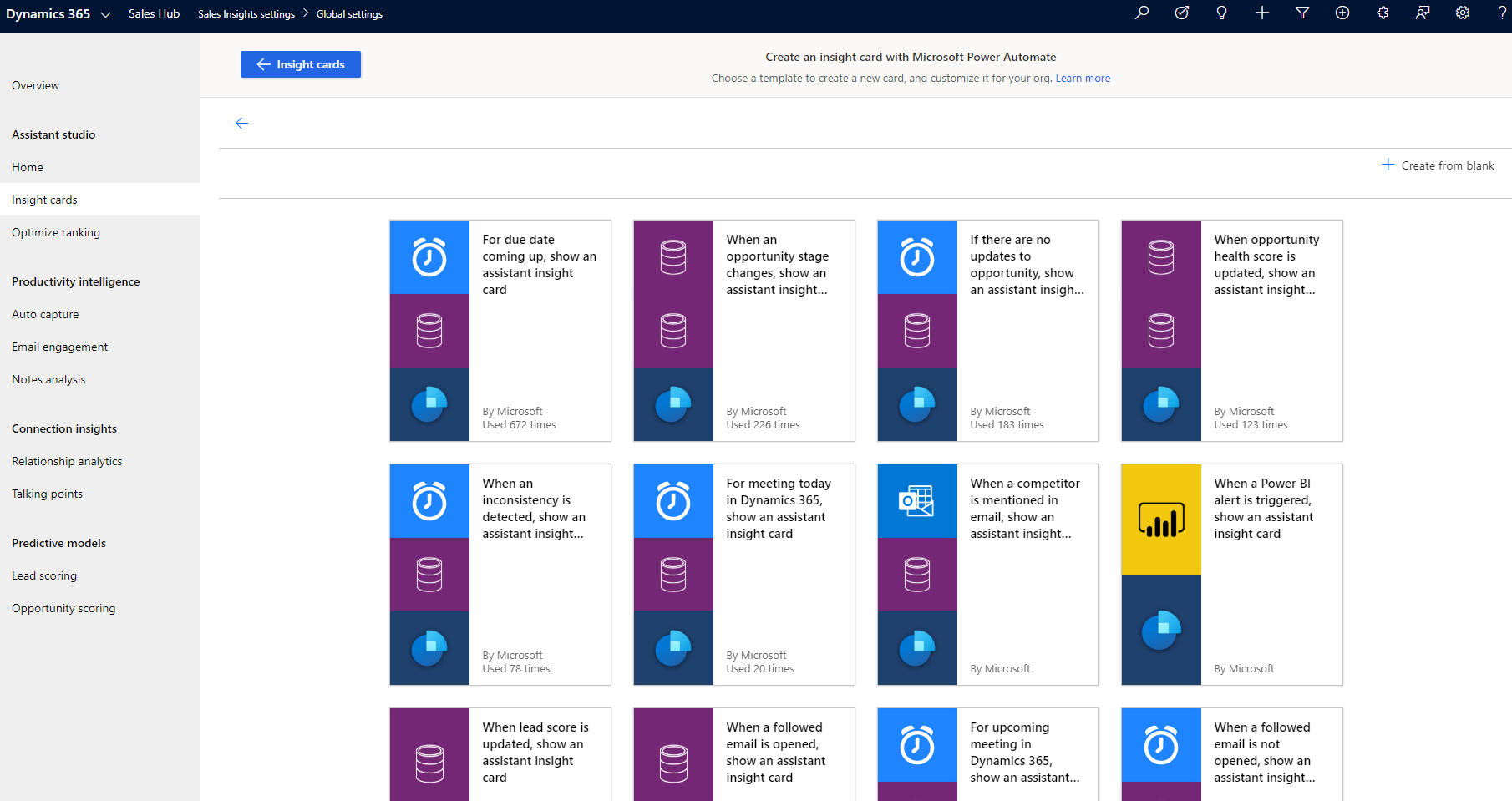In this image, various textual elements and cards are displayed, focusing predominantly on Microsoft's productivity tools and analytics features. On the left side of the image, a vertical list of items is presented, including: Home, Button, Inside Cards, Optimize Ramping, Productivity Intelligence, Auto Capture, Email Engagements, Notes Analysis, Connection Insights, Relationship Analytics, Talking Points, Predictive Models, Lead Scoring, and Opportunity Scoring.

Further, the image elaborates on several specific Assistant Insights cards. Notable entries include:

- "For due date coming up, show an Assistant Insights card." This feature, by Microsoft, has been used 672 times.
- "When an Opportunity Stage changes, show an Assistant Insights card." This is also provided by Microsoft and has been utilized 226 times.
  
Other notable cards in the assortment detail:

- "When Lead Score is updated, show an Assistant Insights card."
- "For upcoming meetings in Dynamics 365, show an Assistant Insights card."
- "When a Powered by Alert is triggered, show an Assistant Insights card."
- "When a Competitor is mentioned in an email, show an Assistant Insights card."

Each of these cards serves a specific function within Dynamics 365, ensuring productivity and insights are optimized for the user.